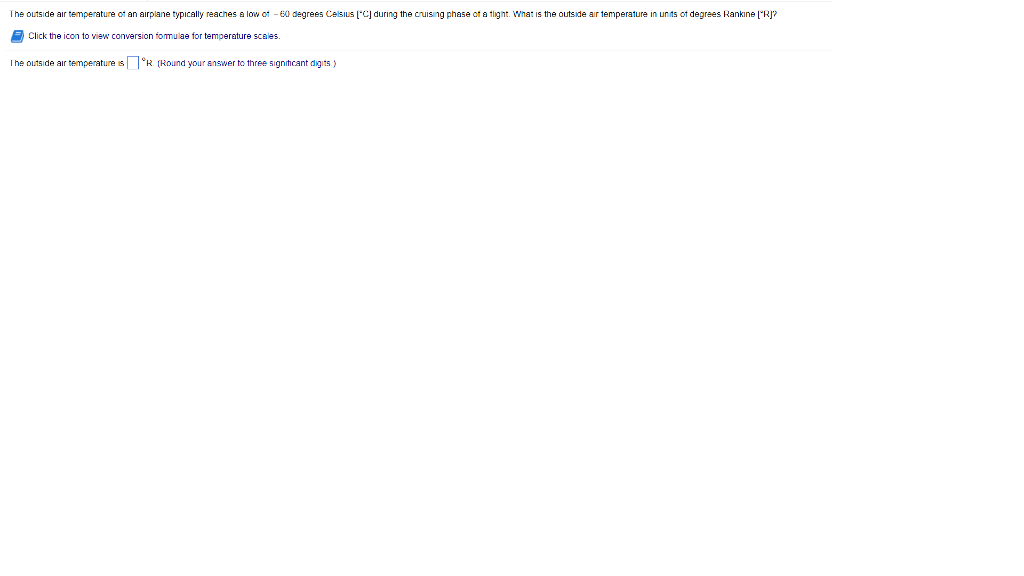This image is a screenshot of an online test question. The incomplete website displays a problem that asks the user to calculate the outside air temperature in degrees Rankine (R) given that the outside air temperature of an airplane typically reaches a low of -60 degrees Celsius during the cruising phase of a flight. The page prompts the user to click an icon resembling a blue book to view the conversion formula for temperature scales. Additionally, it emphasizes rounding the answer to three significant digits. In the top-left corner, directly below the exam question, there are instructions on accessing the conversion formula. The current focus is the problem statement which requires converting -60 degrees Celsius to degrees Rankine.